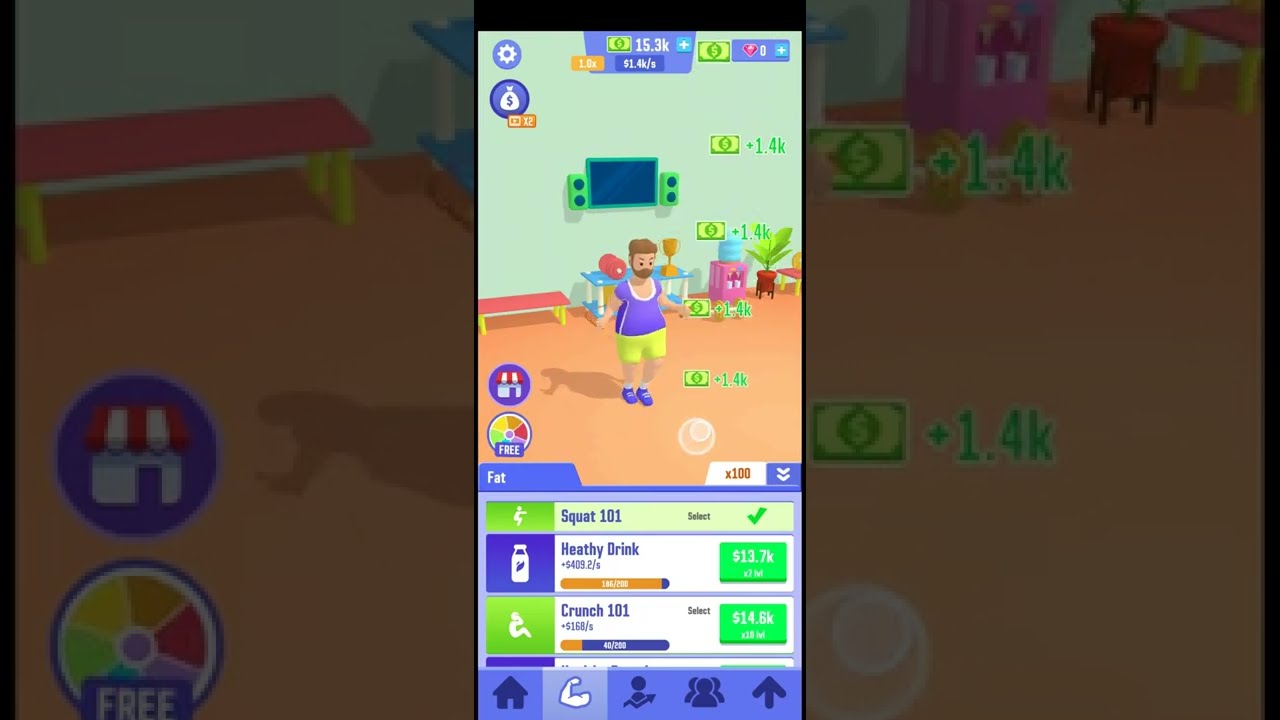The image appears to be a screenshot from a video game, likely an app, featuring a central vertical panel, flanked by two out-of-focus blow-ups of the left and right halves of the main image. In the center of the screen is a cartoon character, a male figure, dressed in a purple tank top, yellow shorts, and purple shoes, standing on an orange floor. The background includes various elements like a green plant in a red planter situated to the right, and a TV behind the character.

The bottom of the screen displays several controls, including icons labeled "squat 101," "healthy drink," and "crunch 101." The "healthy drink" icon is accompanied by a symbol and an orange bar showing a high level, while the "squat 101" icon has a green checkmark next to it. Next to these, there are other indicators and icons, such as a white bottle symbol and an arm flexing.

Monetary details are prominently featured, with green money symbols scattered throughout the screen. The character has accumulated 1.4k in total money, displayed multiple times, with a grand total of 15.3k shown at the top-center of the screen and a money bag icon in the upper left corner. Additional objects in the scene, like a barbell, a table with a water cooler, a trophy, a radio, and multiple benches, are also visible.

The left blow-up of the image shows a cottage with a red striped roof and white walls, while the right blow-up highlights various items like a water cooler and some benches, providing a magnified look at the surroundings. Main colors in the image include green, orange, purple, white, and blue.